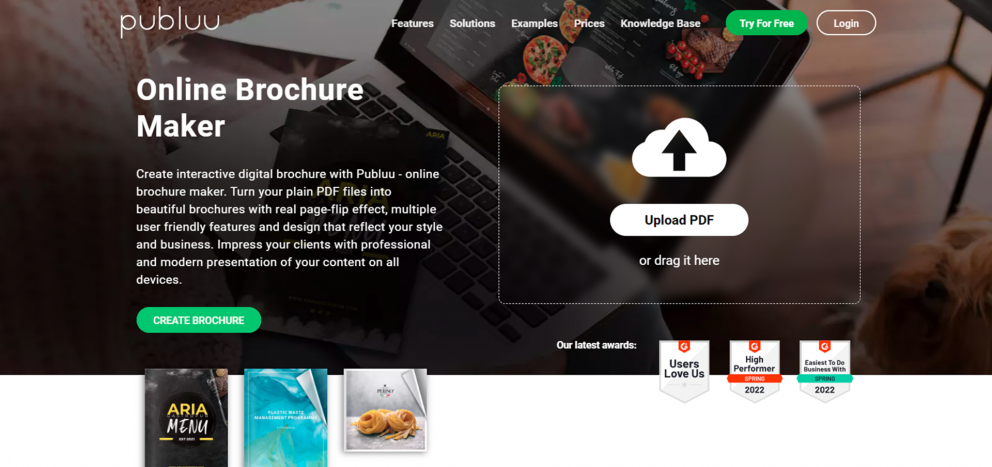The image depicts a screenshot of a website or software interface designed for creating digital brochures. The background features a laptop displaying the website's main page. At the top, white letters spell out "Publuu," which appears to be the name of the service. The tagline beneath the logo reads, "Online Brochure Maker," indicating the primary function of the site.

The page further elaborates with the text: "Create interactive digital brochures with Publuu online brochure maker. Turn your plain PDF files into beautiful brochures with a real page-flip effect, multiple user-friendly features, and designs that reflect your style and business. Impress your clients with professional and modern presentations of your content on all devices."

Below this text, there is a prominent green button with white letters that says "Create Brochure." To the right of this button, a large box features a cloud icon with a black arrow pointing upwards. This box is accompanied by the instructions "Upload PDF or drag it here," suggesting that users can easily start their brochure projects by uploading their PDF files.